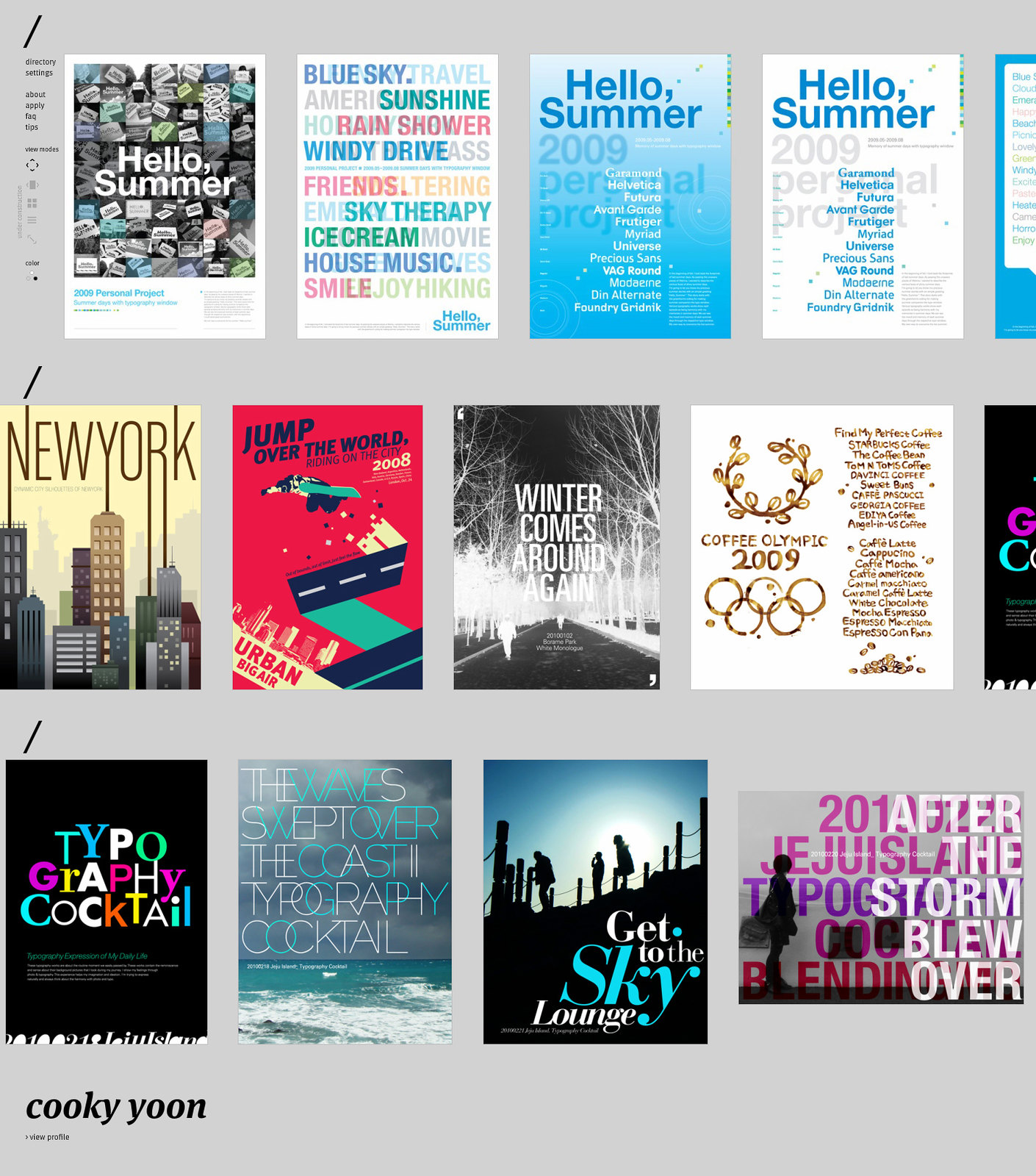The image showcases a gray-background internet browsing page, displaying a detailed array of posters or magazine covers organized into three rows of four columns each. In the top left corner of the page, there's a navigation menu that includes options like Directory, Settings, Apply, FAQ, and Tips. The page provides multiple viewing modes, such as expanding an image, single view, four-per-page view, listing view, and options to zoom and adjust colors.

Each poster on the page is meticulously titled, offering a peek into different themes. The top row features posters with variations of "Hello Summer," including versions labeled "Hello Summer 2009" on both blue and white backgrounds. The second row includes posters titled: "New York," "Jump Over the World," "Winter Comes Around Again," and "Coffee Olympic 2009." The titles in the third row read: "Typography Cocktail," "The Waves Sweep Over the Coast, Morphe Cocktail," "Get to the Sky Lounge," and an incomplete title which appears to end in "2010022." 

In the bottom left corner of the page, there's the name "Cookie Yoon" in a clickable profile link, though additional text below the name is too small to decipher. The overall layout not only highlights the diverse themes of the posters but also emphasizes their vibrant color contrasts designed to catch the viewer's eye.